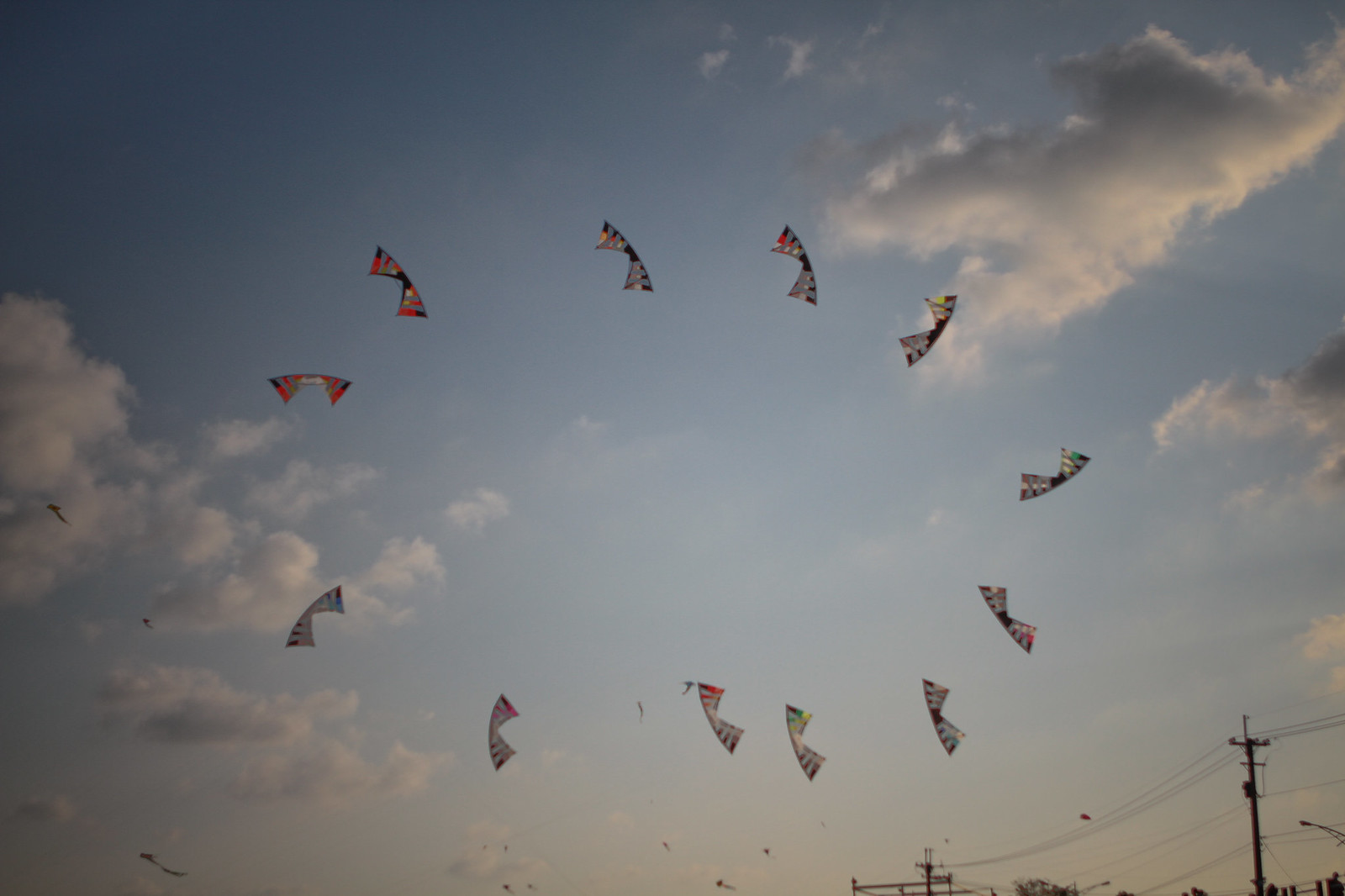This color photograph, shot in landscape mode, features a vibrant blue sky dotted with a few puffy, white clouds mostly concentrated towards the bottom left and top right corners. Dominating the central view, a group of approximately twelve kites, forming an elegant circular pattern, soar high. These kites display an array of colors, primarily black, red, and white, with some featuring streaks of yellow, arranged in almost bow-tie shapes. The photograph captures the scene from the ground looking straight up, creating a sense of upward expanse. In the background, some birds are faintly visible, adding a dynamic touch to the serene sky. Towards the bottom of the image, two telephone poles with cables stretched between them can be seen, grounding the otherwise airy and whimsical composition.